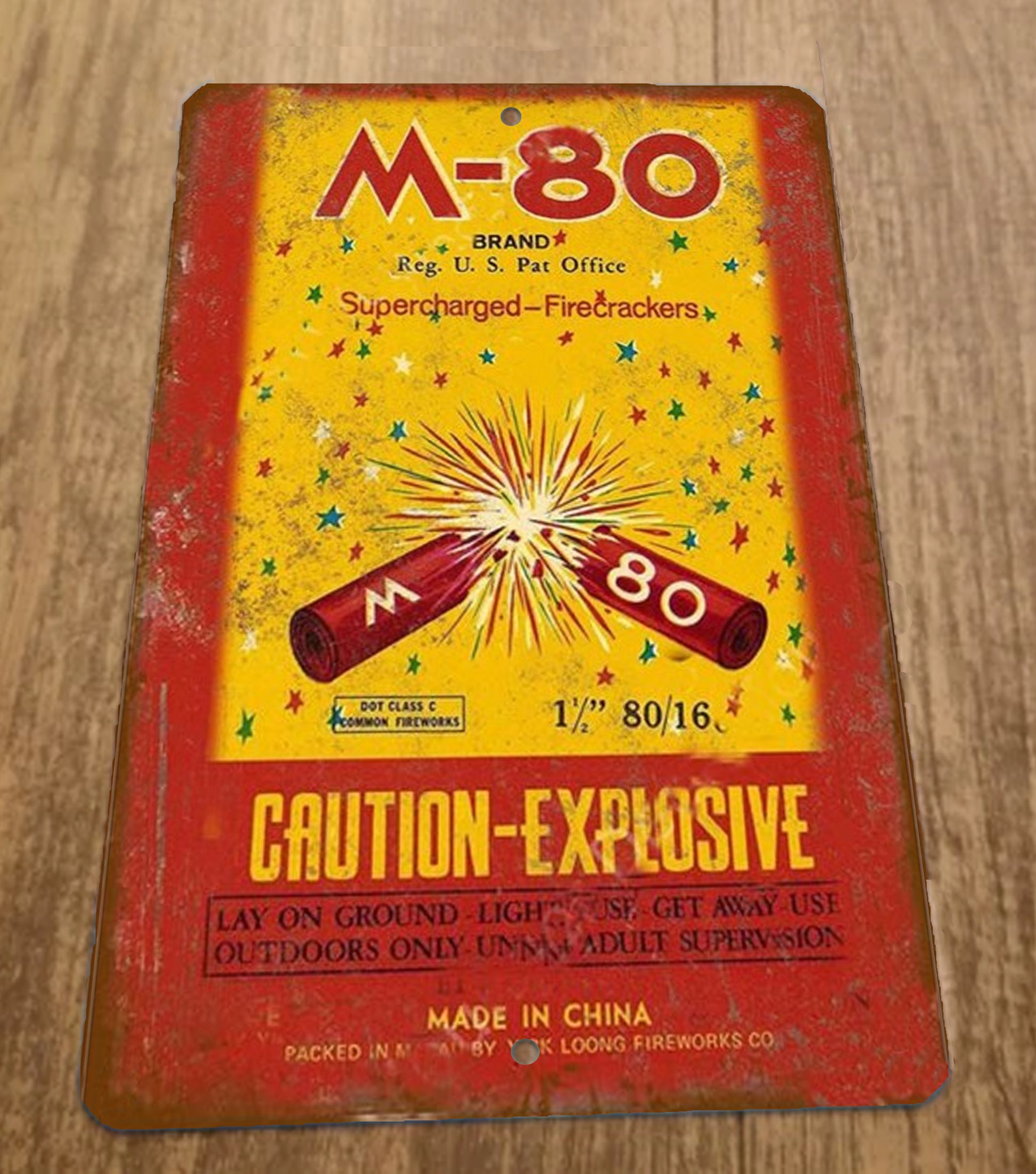The image captures a vintage, worn tin container of M-80 Supercharged Firecrackers, sitting on a rustic wooden surface, possibly a picnic table or an indoor wooden bench. The predominantly red container features a large yellow label across its front. In bold red text on the yellow background, it reads "M-80," and underneath in blue text, "Brand Regulated U.S. Patent Office," followed by "Supercharged Firecrackers" in red. Adorning the label are numerous colorful stars—red, white, blue, green, and yellow—emanating from illustrations of two red firecrackers. The firecracker on the left is marked with an "M" and the one on the right with "80," both emitting visible sparks. Additional text includes "Dot Class C," "1 and a half inches," "80-16," highlighted in red and yellow, and prominently below, the caution message reads: "Caution-Explosives. Lay on Ground, Light, Use, Get Away, Use Outdoors Only, with Adult Supervision" in black text, with "Made in China" noted at the bottom. The packaging has a nostalgic, aged appearance, adding to its vintage charm.